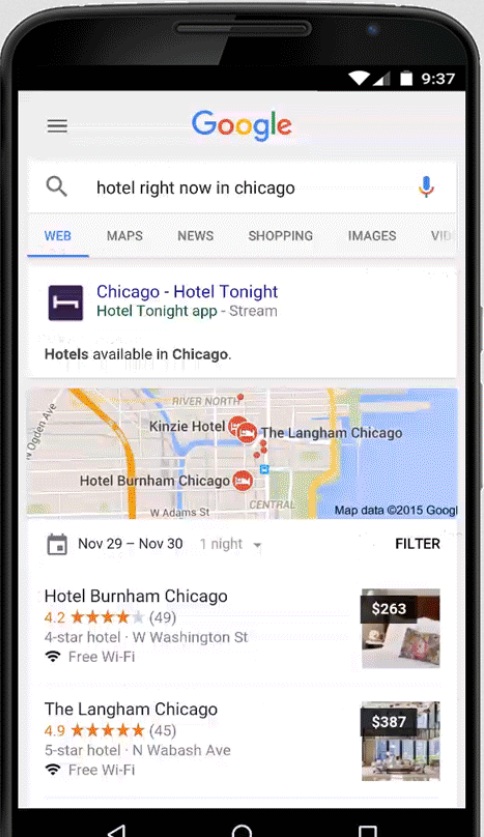This image depicts a meticulously edited screenshot of a mobile phone, showcasing a Google search interface. The phone is characterized by its black bezels, with a solid black status bar at the top. On the right side of the status bar, in white icons, are indicators for Wi-Fi signal, mobile signal, battery status, and the time, which reads 9:37.

Directly beneath the status bar, the phone's screen displays a Google search page that has been altered via photo-editing software. At the upper part of the screen, there is a gray bar with three horizontal black lines in the top left corner, arranged in a vertical stack. Centrally positioned within the gray bar is the Google logo, featuring its recognizable multicolored letters.

Below this, a white search field contains the text "hotel right now in Chicago." To the left inside the search field is a black magnifying glass icon, while on the right side is a blue microphone icon. Underneath the search field, there are search category options listed in a dark gray font: web, maps, news, shopping, images, and video. The "web" option is highlighted, indicating it has been selected.

Proceeding further down, a white rectangular section contains a search result. In the upper left corner of this section is a blue box featuring a white bed icon. Directly to the right is the text "Chicago Hotel tonight," displayed in a blue font.